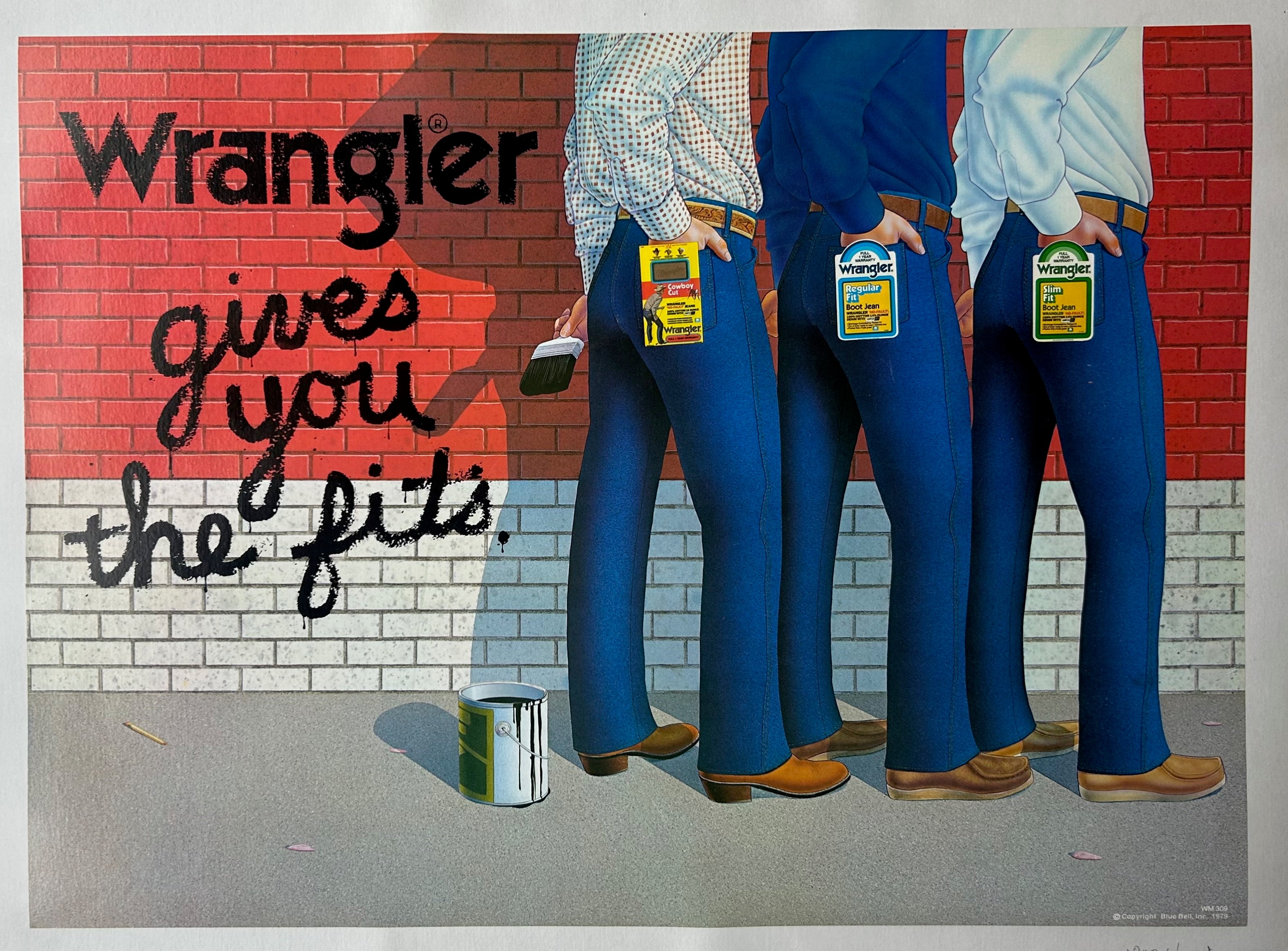This color print advertisement for Wrangler is a detailed illustration that features three men standing side by side against a brick wall background. The top half of the wall is red, while the bottom half is white. Written prominently on the wall is the slogan "Wrangler gives you the fits." The men are depicted from the chest down, each dressed in distinct outfits but uniformly wearing Wrangler jeans with labels on the back pockets indicating the different fits: Cowboy Cut, Regular Fit Boot Jean, and Slim Fit Boot Jean. 

The first man, clad in a checkered long-sleeve shirt, brown belt, and brown shoes, holds a paintbrush behind him, with a can of black paint on the ground nearby. The second man sports a blue denim shirt paired with dark loafers, while the third man wears a gray shirt and brown loafers. All three men have their right hands in the back pockets of their jeans. Each label and tag highlights the variety Wrangler offers, enhancing the impact of the advertisement while keeping the viewer's focus on their jeans. The image is copyrighted by Bluebell Inc. 1975.